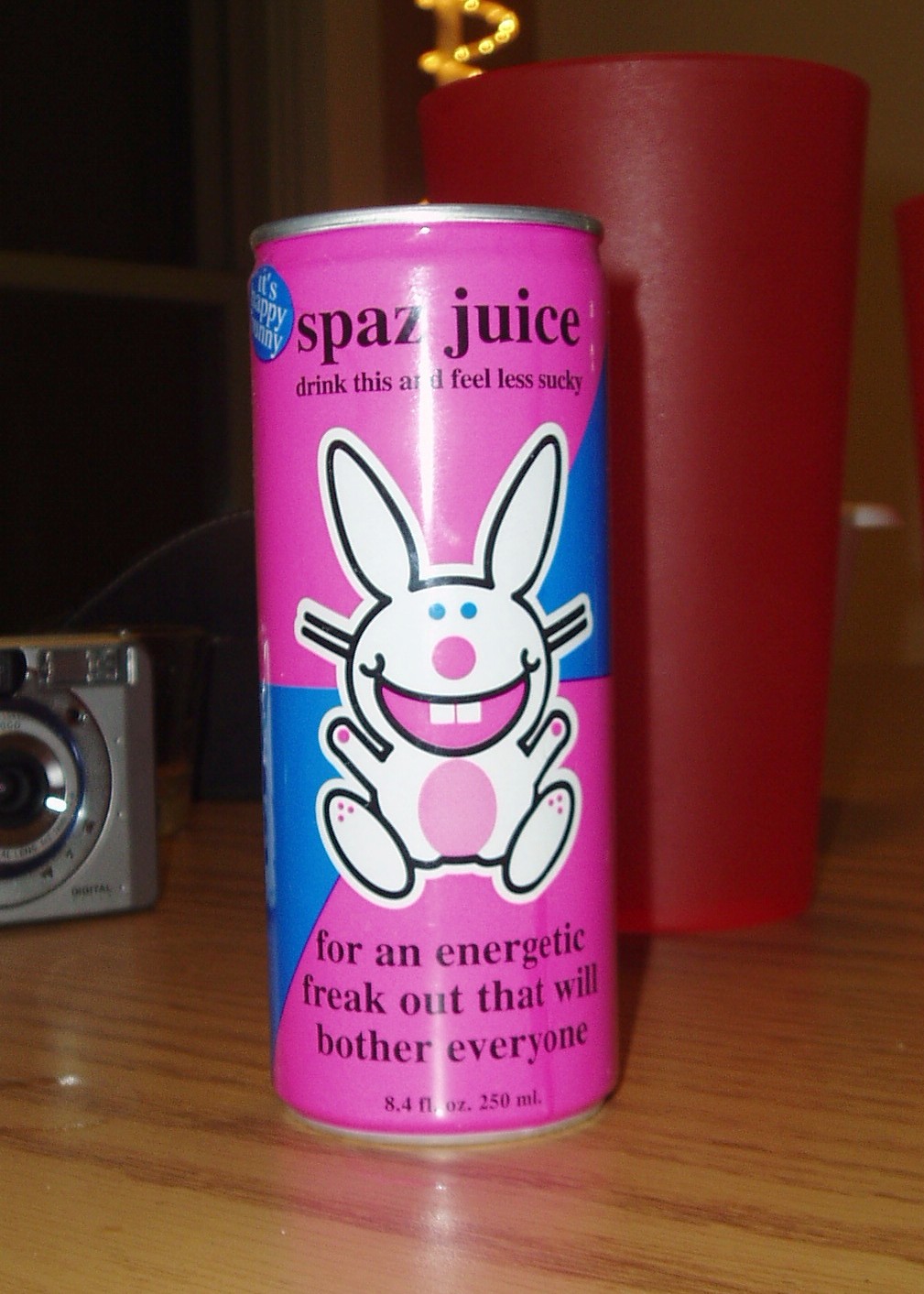The image features a vibrant aluminum can of "Spaz Juice," an energy drink. The can, predominantly pink with blue accents, showcases a cheerful white bunny with blue eyes, a pink nose, a pink mouth, and two prominent white teeth. The bunny, depicted with pink pads on its feet and pink on its torso, is smiling energetically. The text on the can reads, "Spaz juice: Drink this and feel less sucky," followed by, "For an energetic freakout that will bother everyone." The can's capacity is marked as 8.4 fluid ounces (250 milliliters). Positioned on a brown wooden tabletop, the foreground of the image sharply focuses on the can, while the background includes a red plastic cup slightly taller than the can, adorned with a gold symbol at its top. To the left of the can is a partially visible old-fashioned digital camera with a noticeable silver lens, adding a touch of retro flair to the setting.